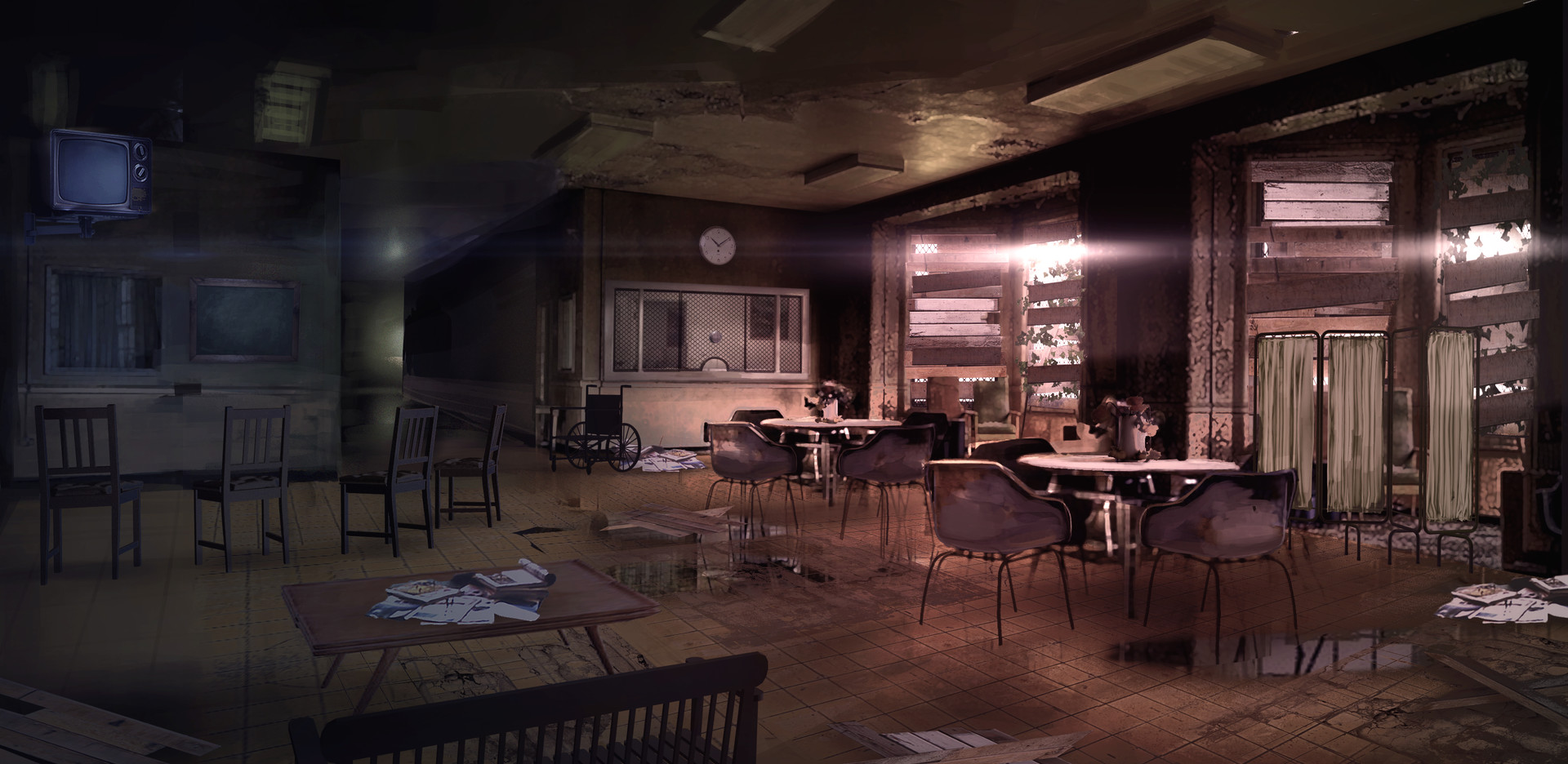The image captures the interior of an obviously abandoned and possibly old library or office space. The floor is coated in copper-colored tiles, while natural light seeps in through partially boarded-up windows, casting an eerie glow across the room. The right side of the scene is illuminated, but for the most part, the space remains dim and gloomy. 

On the left side, a sturdy wooden table accompanied by numerous wooden chairs stands prominently, alongside another smaller table with a wooden bench in front of it. Further back, round tables surrounded by chairs are visible. In the background, a clock adorns the wall above a large window that features a steel sliding door. Amidst the arrangement, a lone wheelchair hints at a once-functional space, while some portable curtains to the right suggest it might have served a medical purpose. Scattered papers on some tables further attest to the building's dilapidation. The overall imagery conveys a poignant sense of desolation and neglect within this spacious, once-active facility.